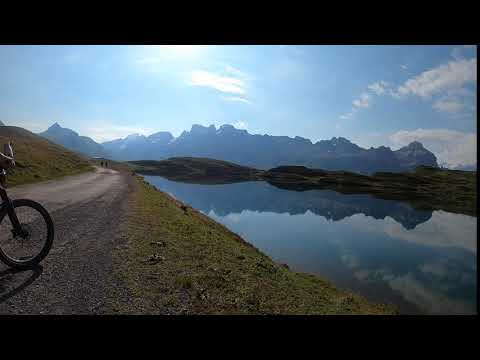The image showcases a serene black sand beach with a clear, reflective body of water. The scene is bordered by thick black lines at the top and bottom. To the left, a brownish, dark gray road or path inclines gently toward the water. In the foreground, the front wheel of a bicycle and an owner's hand on the handlebar are visible, suggesting someone has stopped to take in the idyllic view. The path is flanked by short grass leading down to the tranquil, wave-free water. The water's surface mirrors the blue sky dotted with a few scattered clouds, and the imposing mountain range in the background. The reflection includes the mountains, sky, and nearby rocks, adding depth to the scene. Additionally, two tiny black lines far back on the path might be distant figures, adding a sense of scale and distance to the picturesque landscape.